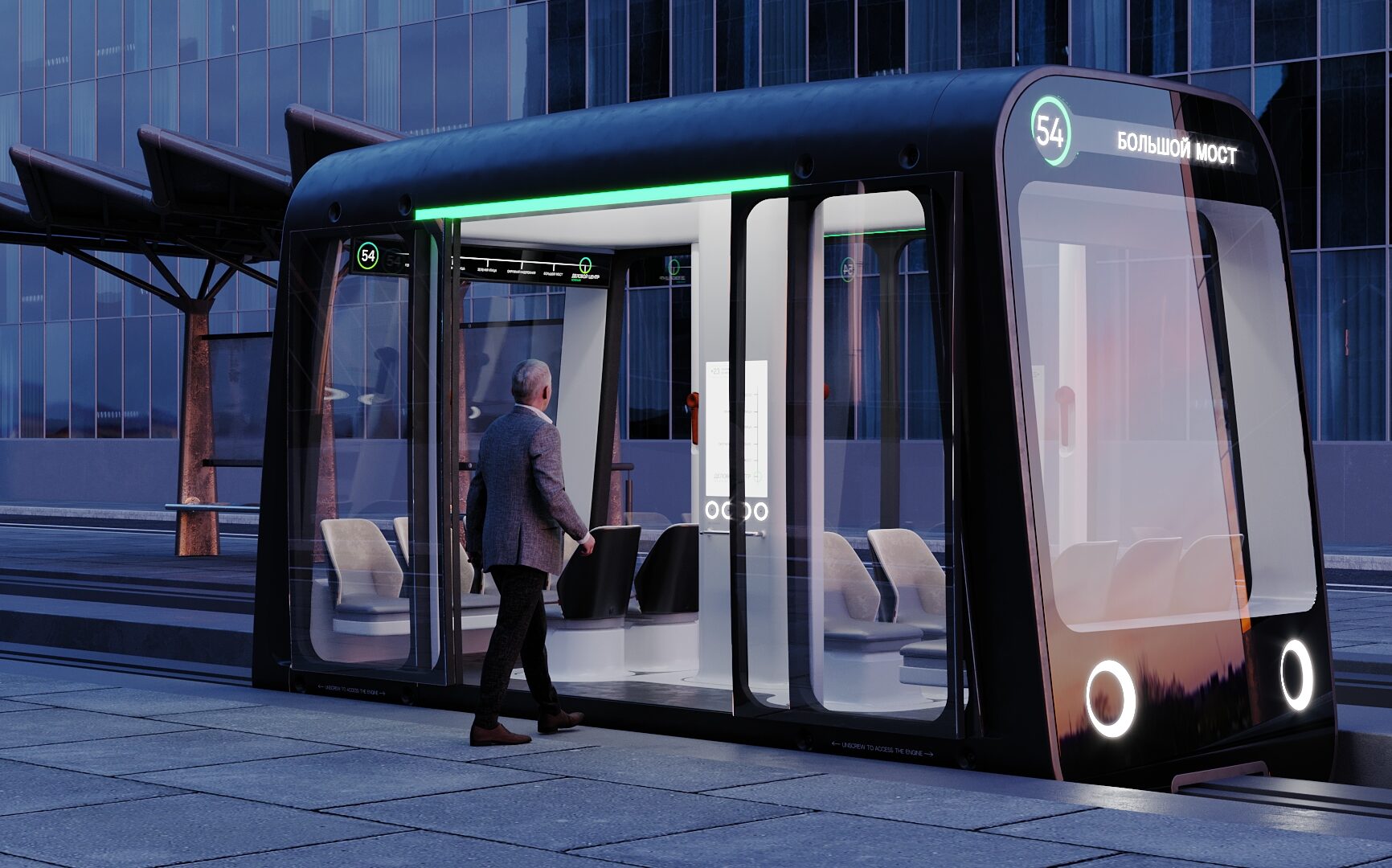The image depicts a highly detailed artist's concept rendering of an autonomous monorail shuttle at a modern railway platform. The monorail, designated with the number 54 and featuring non-English text at its front, is a sleek vehicle with a dark purple and black exterior. Its front is equipped with two circular headlights. The shuttle, currently at a stop, has its door open with a man walking towards it, clad in a gray jacket and black pants. The interior of the monorail is well-lit, revealing multiple rows of seats in black and gray. The platform itself is composed of rectangular gray tiles. In the background, there are several towering high-rise buildings, characterized by their blue-tinted glass facades, adding to the modern and futuristic ambiance of the scene.